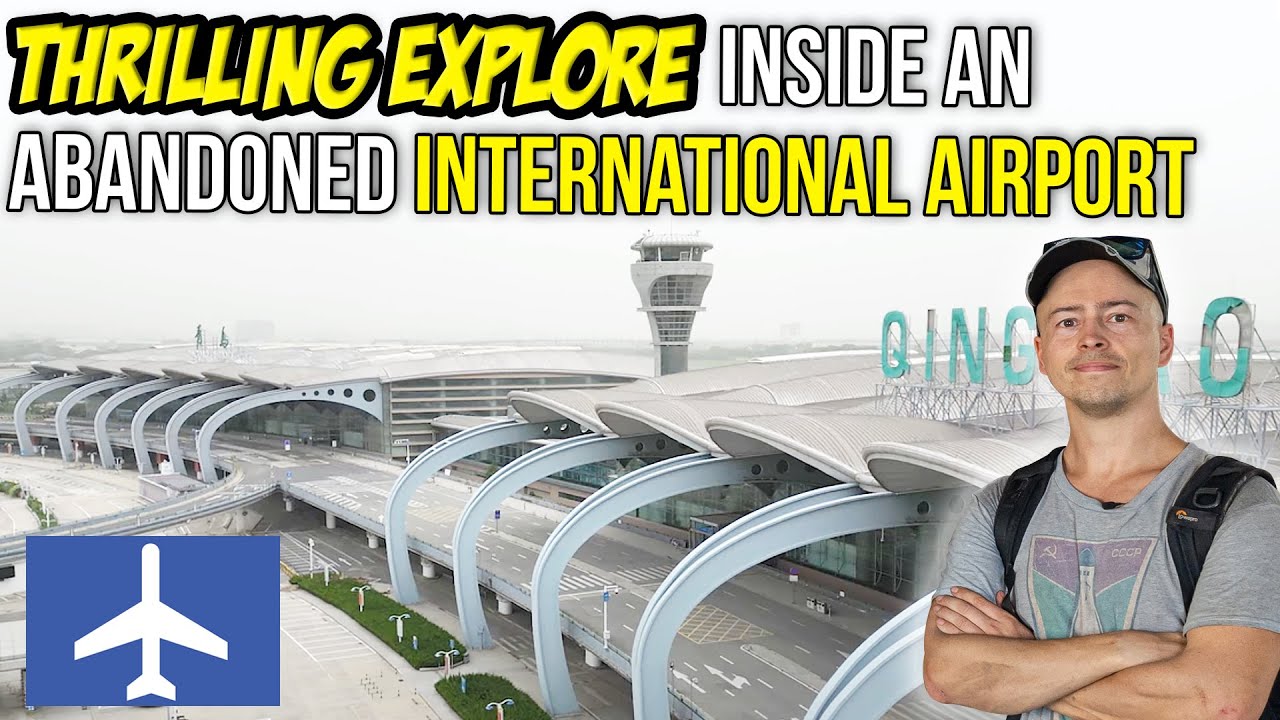This image appears to be a title card for a YouTube video or similar, featuring a promotional shot for a video titled "Thrilling Explore Inside an Abandoned International Airport." The text spans the top of the image in capital letters, with "Thrilling Explore" and "International Airport" highlighted in yellow, while "Inside" and "Abandoned" are in white, all outlined in black.

The background showcases an exterior view of a modern, slightly dilapidated airport, with visible arched silver supports extending over a multi-laned driveway. A partially obscured light blue sign reads "QING...O," and there's a prominent air traffic control tower in the scene. In the bottom right corner stands a man, presumably the explorer or tour guide, with a stern expression, his mouth closed and arms crossed. He wears a gray t-shirt with some red and green design, a black backpack, and a tan baseball cap with sunglasses perched on top. He appears to be in his middle age, sporting a partially shaven look.

On the bottom left of the image, there's a blue rectangle featuring a white airplane icon, reinforcing the aviation theme. Overall, the image combines elements of text and visual details to create a dramatic and engaging advertisement for an exploration video set in an abandoned international airport.